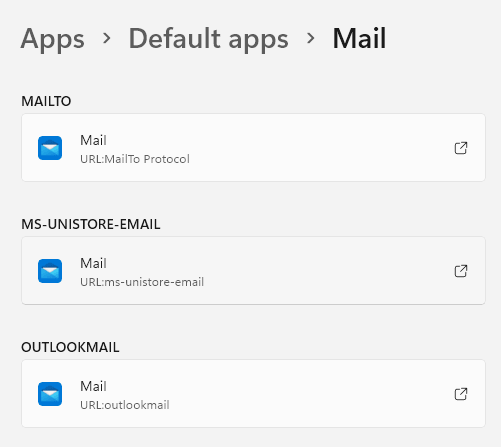This image displays a detailed interface specific to configuring mail settings. At the top, the navigation path is highlighted in a clear, large black font, beginning with "Apps," followed by a right-pointing arrow, then "Default Apps," another right-pointing arrow, and finally "Mail." The capitalized letters in "Apps," "Default Apps," and "Mail" indicate the hierarchy and focus of the page, with "Mail" in a darker black to emphasize the current section.

Below this navigational path, there is a spaced section featuring three labeled boxes for configuring different mail protocols. Each label is left-justified. The first box is labeled "Mail to," associated with a white box containing the URL "mailto protocol." The second box is labeled "Unistore mail" with the URL "ms-unistore-mail." The third box is labeled "Outlook mail," where its associated white box displays the URL "Outlook mail." This structured arrangement aids in adjusting settings for various mail applications within the interface.